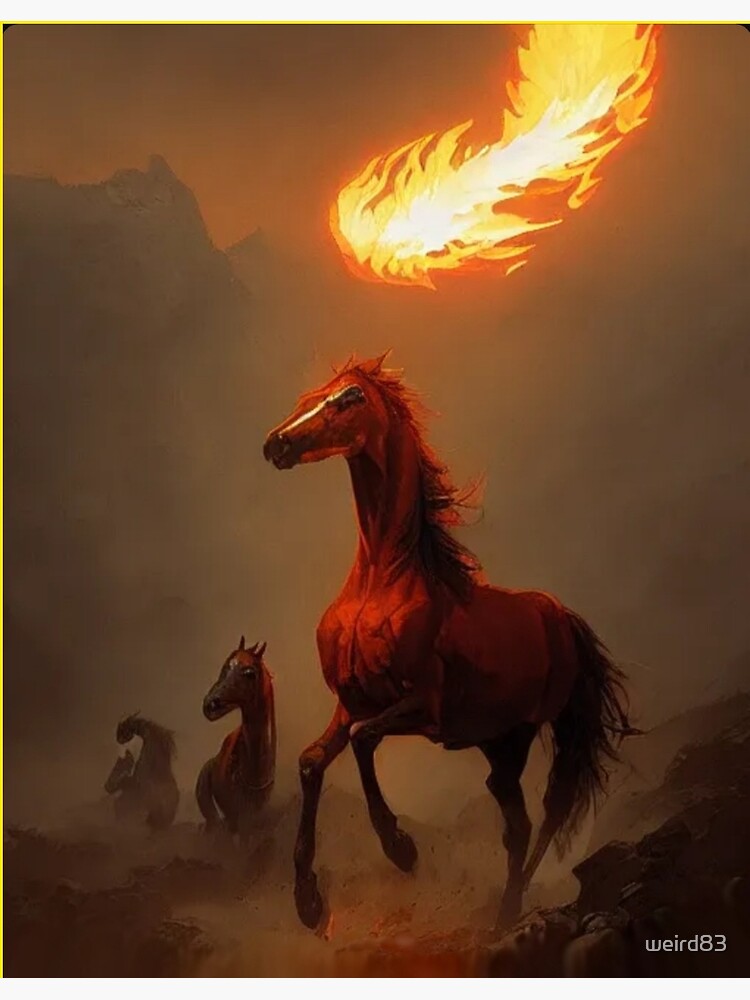This striking piece of original artwork captures a surreal and intense scene featuring three animated or illustrated horses in a smoky, fiery environment. The prominent foreground features a large red horse walking through a landscape filled with rubble and potential blood, with its expression hinting at urgency. The background includes two smaller horses, which appear to be either running or galloping away, rendered in a manner that gives a sense of depth and perspective. 

The entire scene is engulfed in a thick, smoky atmosphere with a massive flame rising from the top of one of the distant mountains, cutting off at the top edge of the image. The sky above transitions into hues of dusky amber and blackish orange, filled with ash and smoke. Rocky outcroppings and shadowy mountains lend a grayish tone to the backdrop, further emphasizing the devastation. 

Interestingly, a small dragon is subtly included in the background, looking back over its tail, adding a mysterious element to the chaotic environment. 

The artist's signature, "WEIRD 83" in white or grey, is distinctly visible at the bottom right corner, underscoring the uniqueness and originality of the piece.